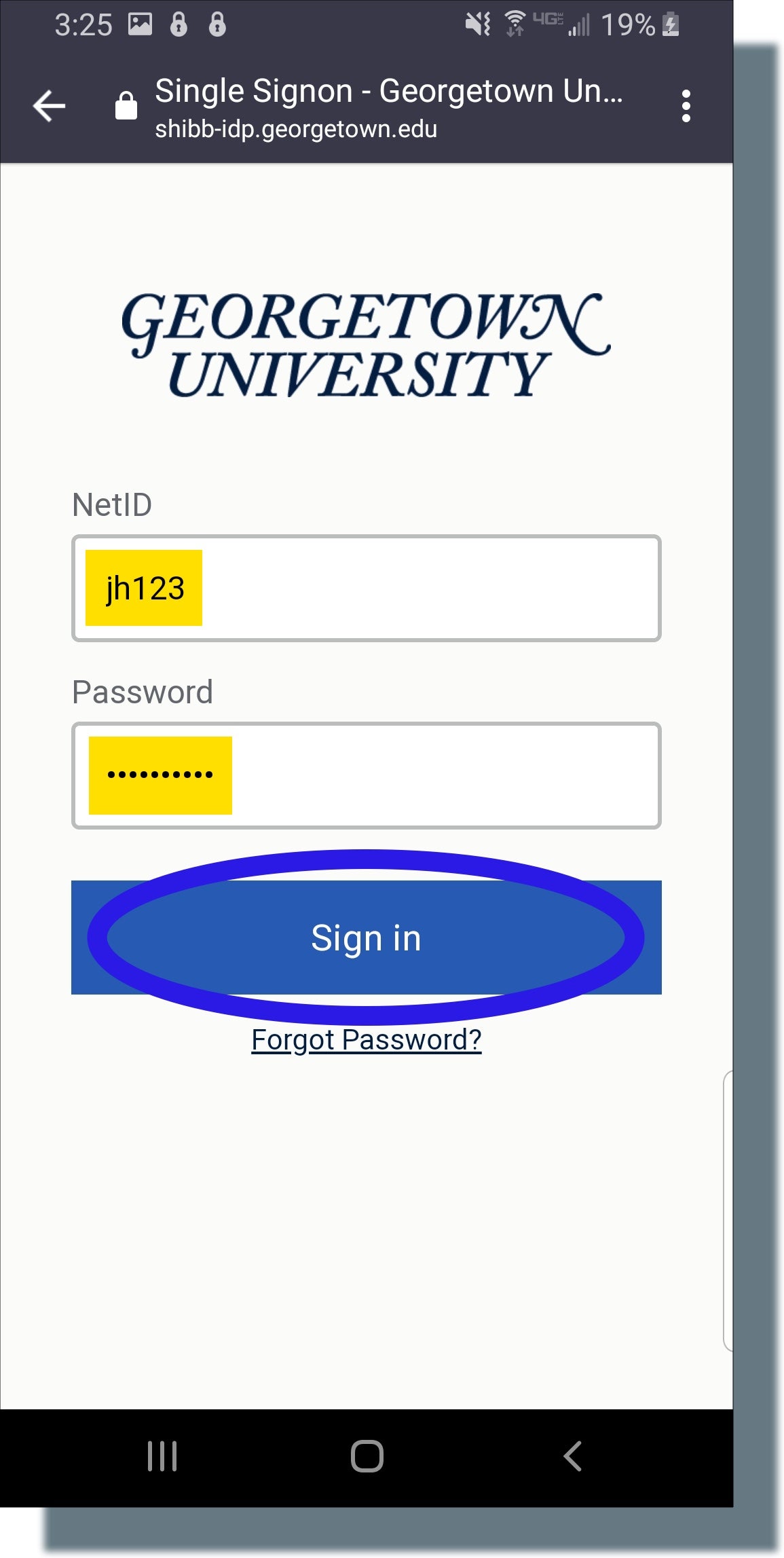The image shows a smartphone screen displaying a website open at 3:25 PM, as indicated by the time icon on the top left of the screen. Other icons on the top left include a screenshot icon and two lock icons. On the top right of the screen, additional icons appear, including a 19% battery icon, Wi-Fi icon, and two news icons.

The website displayed is the Single Sign-On page for Georgetown University. The background is dark with white text and icons. The website URL shown is shibidp.georgetown.edu. Below that, the background switches to white, featuring the text "Georgetown University" in dark purple. 

Further down, the page prompts for a "NetID" with a corresponding text box. Inside the text box, the ID "JH123" is written in black. The background where the text appears is yellow. Below the NetID section, there’s a password input field with black dots obscuring the password for security. The background for this input field is also yellow.

At the bottom of the form, there is a "Sign In" button with white text on a blue background. An annotation circle highlights the "Sign In" button, with the circle matching the blue of the button. Below the button, "Forgot Password" is written in dark blue.